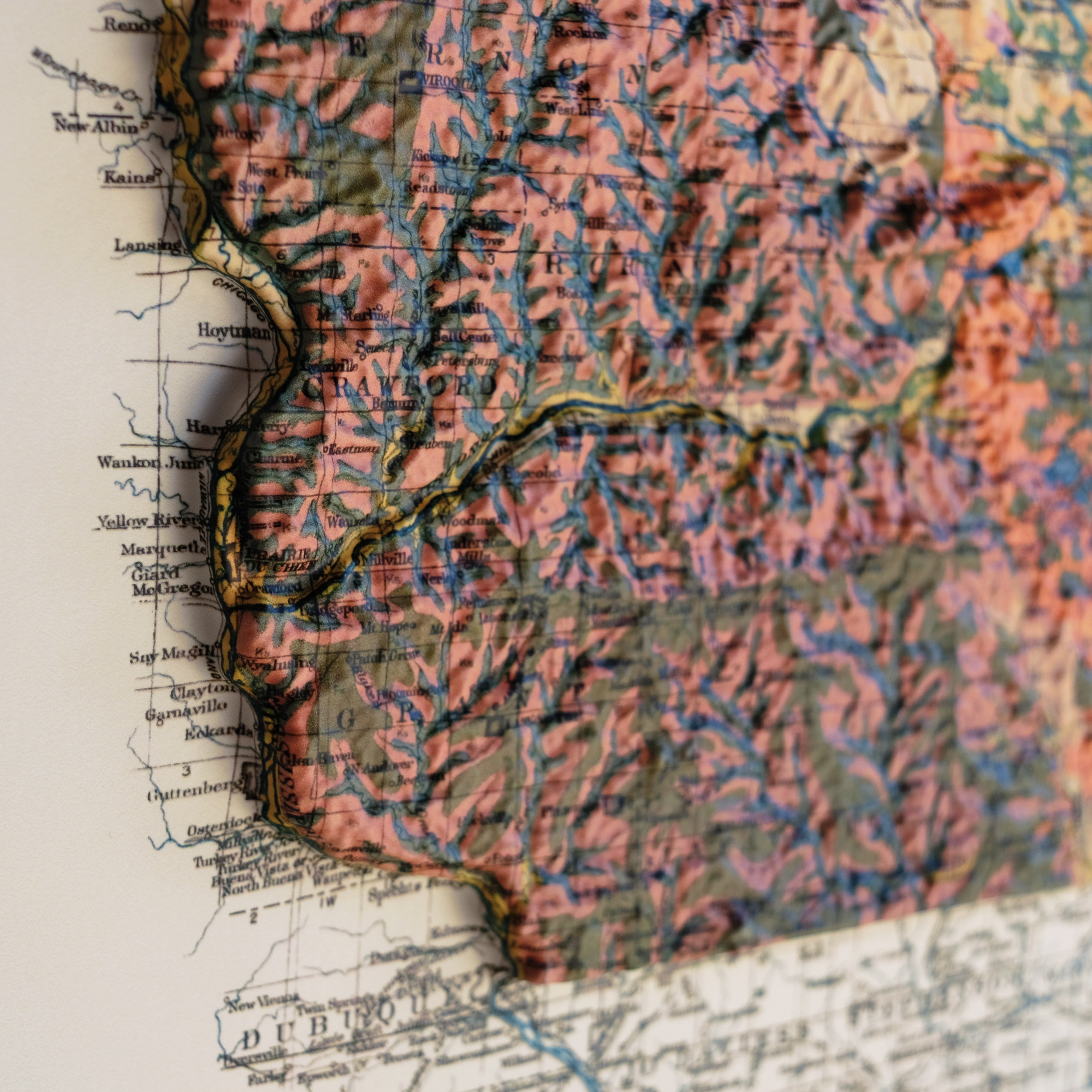The image showcases a detailed, three-dimensional topographical map overlaying a traditional flat map on an off-white background. This layered map features prominently raised and indented areas that give it a textured, bumpy feel with noticeable elevation changes representing mountainous regions. Various geographical elements like roads and rivers are visible, with rivers highlighted in blue, resembling veins. The map also features distinctive green and reddish-brown hues, reminiscent of verdant landscapes and red rock formations. Key identifiable labels include "Crawford" on the left side, "ERNON" in the upper left corner, and "DUBUQUE" in the lower left corner, though much of the text remains blurry and indistinct. Covering about three-quarters of the image, the 3D elements make the map appear to float above the base layer, creating an engaging visual depth intended for educational or illustrative purposes.